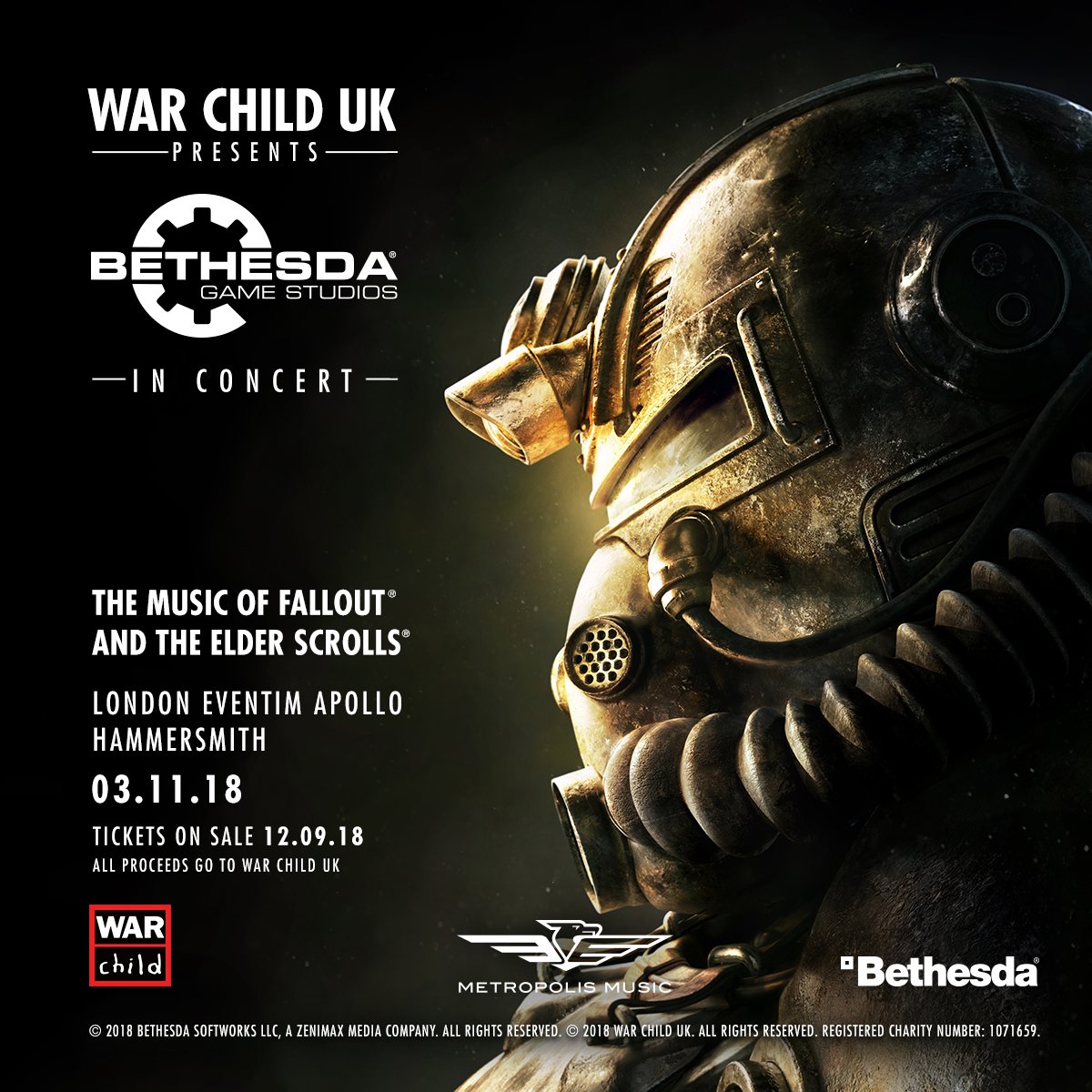This detailed promotional poster for a concert highlights an upcoming event organized by War Child UK, featuring Bethesda Game Studios. Dominated by white capital letters, the top left corner prominently states "War Child UK presents," followed by Bethesda’s iconic logo, a circle with a gear symbol. Below, it announces "Bethesda Game Studios in Concert," the event showcasing "The Music of Fallout and The Elder Scrolls."

Set against a backdrop of mixed hues including white, yellow, brown, a tinge of green, black, and red, the poster details the event location and date: "London, Eventim Apollo Hammersmith - 03.11.18." All proceeds from the concert will support War Child UK, as emphasized by the red-outlined box with the white letters "War" over "Child."

Additionally, there's an illustration of a man in a metal helmet on the right side, facing left. At the bottom center, the sponsors "Metropolis Music" are represented with a bird symbol, while to the right, "Bethesda" is written prominently. Copyright details read: “Copyright 2018, Bethesda Software Works, LLC, a ZeniMax Media Company, All Rights Reserved” and “Copyright 2018, War Child UK, All Rights Reserved, Registered Charity Number 1071659.” 

Key event details include tickets going on sale from December 9th, 2018, further cementing this as a charitable and musically rich event supporting a notable cause.